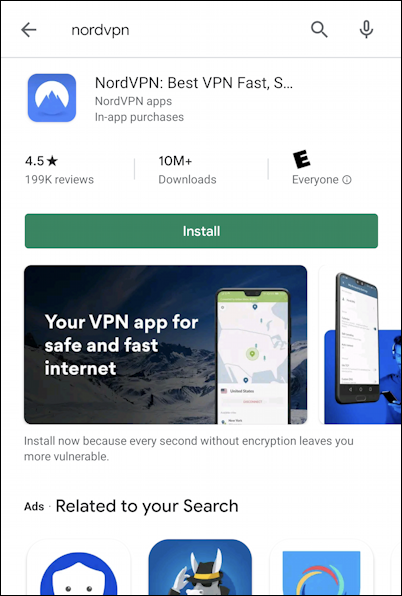This image appears to be a screenshot of a search result for the VPN application "NORD VPN." The app icon features a blue graphic of three mountain peaks—a dominant central peak flanked by two smaller ones—enclosed within a rounded square icon. The icon's background is white. The description for NORD VPN highlights its reputation as the best VPN for fast internet service and mentions that there are in-app purchases available. Impressively, the app has been downloaded over 10 million times and boasts a 4.5-star rating based on 199,000 reviews.

Prominently displayed within the screenshot is a large green rectangular button labeled "INSTALL" in white text. Below this button, there are several promotional images, including one of a mobile phone against the backdrop of a picturesque Swiss Alpine landscape. Superimposed over this scenic image is the text "Your VPN app for safe and fast internet," written in white.